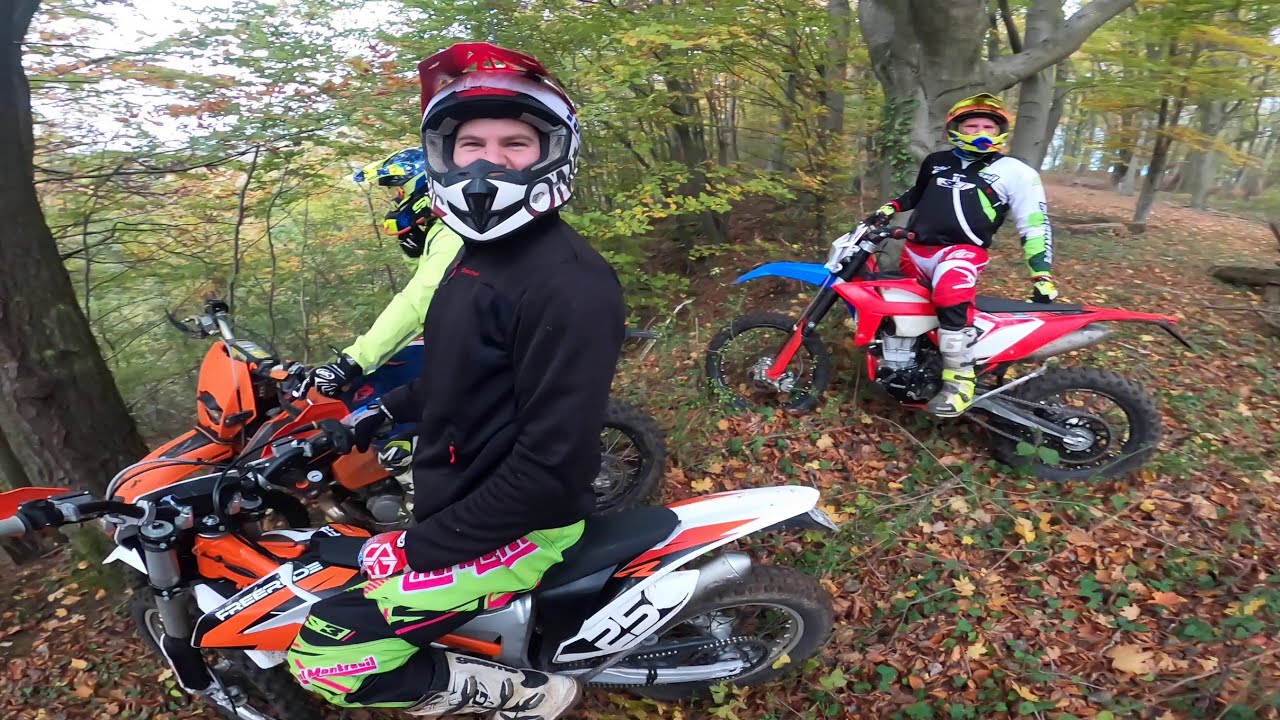In this image, three motorcycle riders are positioned centrally, prominently set against a backdrop of a dense forest. The ground is strewn with leaves, sticks, and brush, indicating it is autumn, as suggested by the vibrant colors of the foliage—shades of brown, red, orange, green, white, black, and blue. The riders, equipped with helmets and full motocross gear, are riding or possibly taking a break on a ledge in the woods, which descends into a canyon filled with a large grove of trees. Two of the riders gaze directly at the camera, while the third looks away. Their dirt bikes are vividly colored: the one in the foreground is white and orange, the one in the middle is black and orange, and the bike in the background is red, white, and blue. The scene is set outdoors in the middle of the day, capturing a moment of adventure amidst nature.